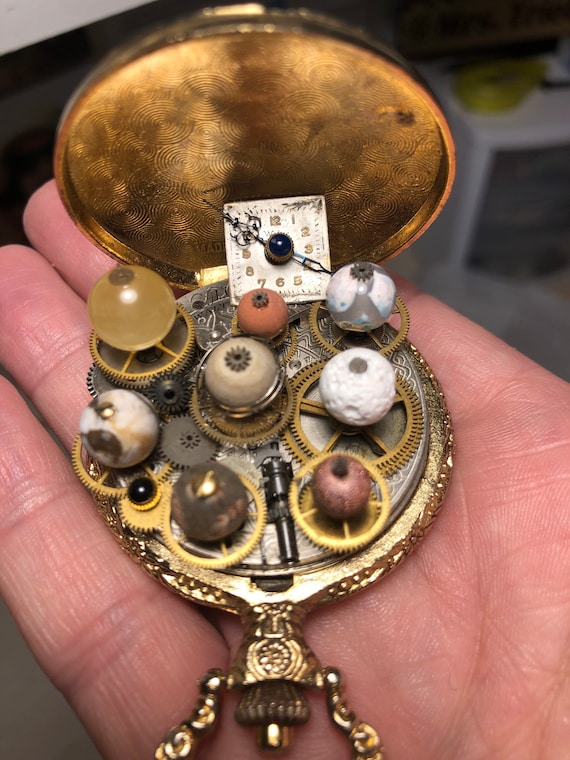In a close-up photograph, a hand with a Caucasian skin tone holds an open gold pocket watch, evocative of a repurposed, artistic creation. The watch's interior is filled with an array of gears, small and large, interspersed with eight polished beads. These beads vary in material; some appear to be glass, others resemble white stone, and a few seem wooden. Each gear incorporates a central sphere, resembling an eyeball or a smooth marble. Leaning against the open lid's top is a small, disconnected watch face with long arms extending beyond its square frame. The overabundance of elements within the pocket watch makes it impossible to close, suggesting it has been reimagined as a piece of intricate art rather than a functional timepiece. The background, though blurred, hints at a possible home or workshop setting.